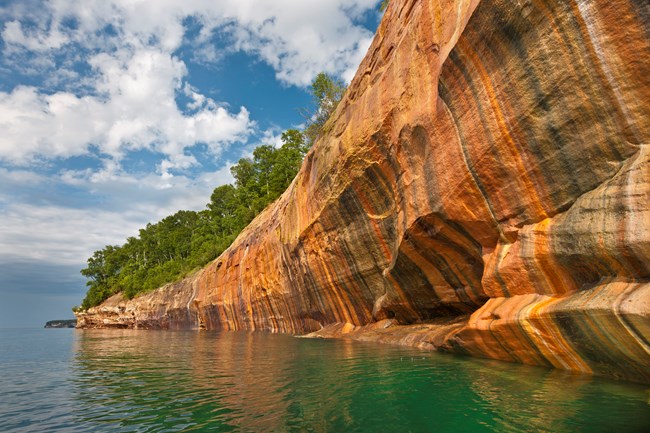This is a photograph capturing a dramatic landscape dominated by a towering rock formation adjacent to a greenish-colored lake. The rock, showcasing vertical striations that create a striking pattern of orange, brown, black, and white layers, takes up the majority of the image. Positioned on the right-hand side, it gradually tapers down towards the left, almost coming to a pointed edge. Atop the rock, lush green trees are visible, reflected in the serene water below. The perspective of the photo is from near water level, looking upwards towards the imposing rock, emphasizing its height and grandeur. The upper part of the photograph features a blue sky dotted with clouds, adding to the natural beauty of the scene.